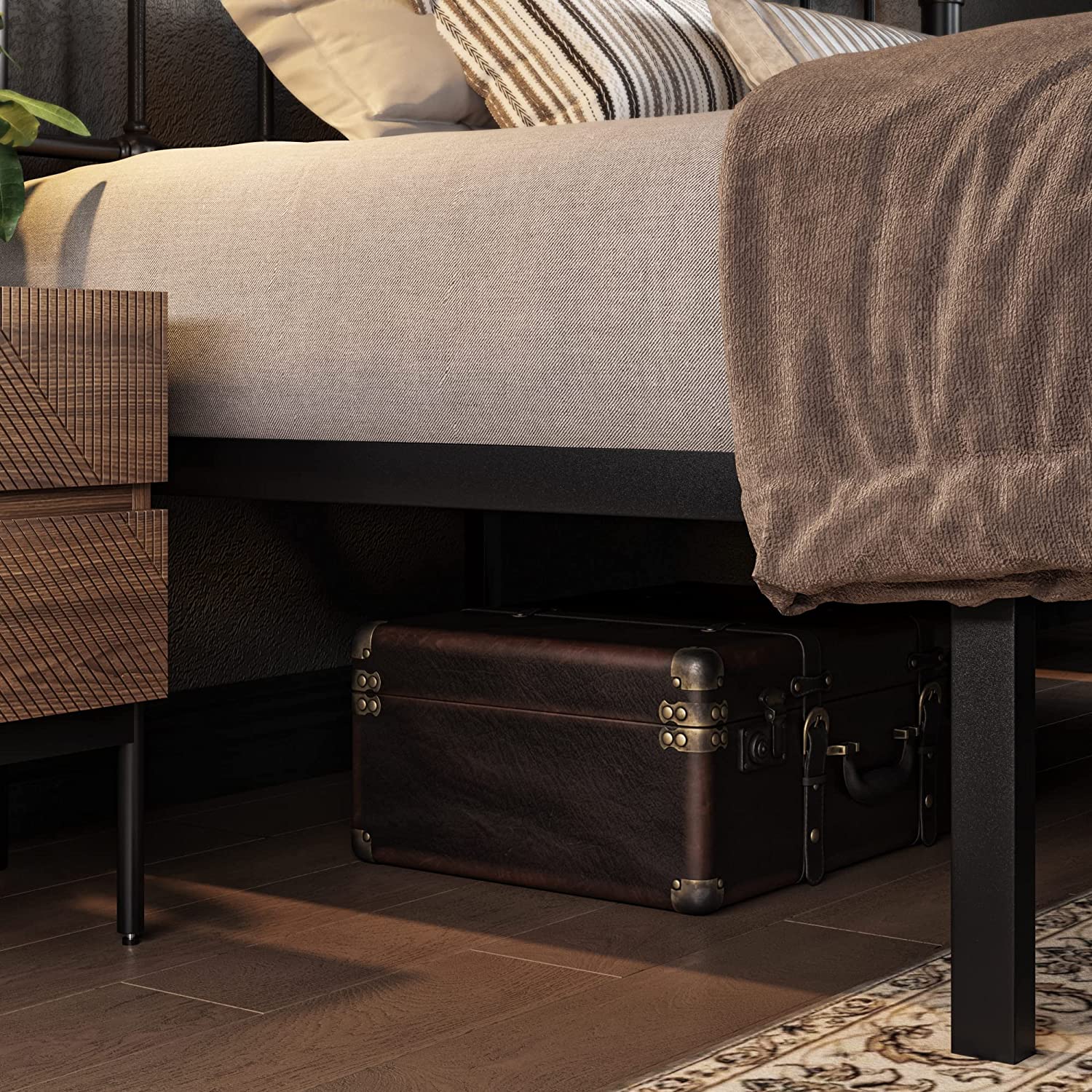This detailed photograph captures the side view of a bedroom, focusing primarily on the area under an elegantly styled bed. The bed features a black metal frame and a matching metal headboard, of which only two horizontal rungs are peeking out from behind the pillows. The beige-colored bed covering is pulled back just enough to reveal a brown suitcase resting under the bed. The mattress is adorned with off-white sheets and topped with three pillows: a plain beige one at the back, followed by two pillows with beige backgrounds adorned with gray and brown stripes on their pillowcases. The blanket draped over the bed is a rich brown color, folded neatly.

To the left side of the bed, there is a rattan and metal bedside table, partially visible, with just a hint of its legs in the frame. Atop the table sits a green plant, with only a couple of leaf tips evident in the photograph. The floor beneath the bed is a mixture of wide wooden planks with a light brown finish and a tan and beige carpet. The overall flooring seems reflective, adding a touch of shine to the light brown wooden surface. The photograph also captures a fragmented view of a beige and brown oriental rug in the right-hand corner of the room and emphasizes the cozy, coordinated color palette throughout the bedroom.